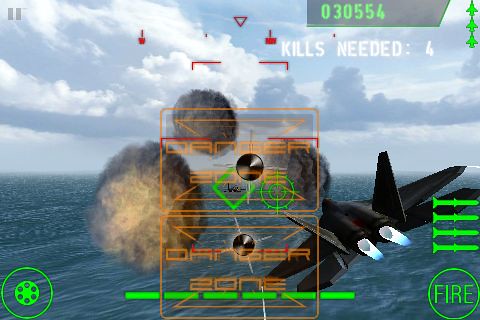In this computer game scene, the viewer is presented with a vivid depiction of aerial combat set against a serene backdrop. The sky is a clear blue, dotted with fluffy white clouds, conveying the sense of high altitude. In the upper right-hand corner of the screen, a gray bar displays green numbers reading "030554", with a small indicator below in white font stating "Kills Needed: 4".

Dominating the foreground, a sleek black airplane is in motion, flying over a vast expanse of water. Bright blue flames, possibly from afterburners, are visible trailing from the plane's engines, adding to the dramatic sense of movement and urgency. In addition, three gray explosions or bomb blasts are seen in front of the airplane, heightening the chaotic atmosphere of the scene.

To the right of the plane, a clear box outlined in orange contains strategic numerical data crucial for gameplay. Additionally, in the bottom right-hand corner, a circular icon displays the word "Fire" in bold green letters, suggesting a control mechanism or an indication of remaining firepower. The ensemble of these elements creates an engaging and dynamic snapshot of an intense moment within the game.